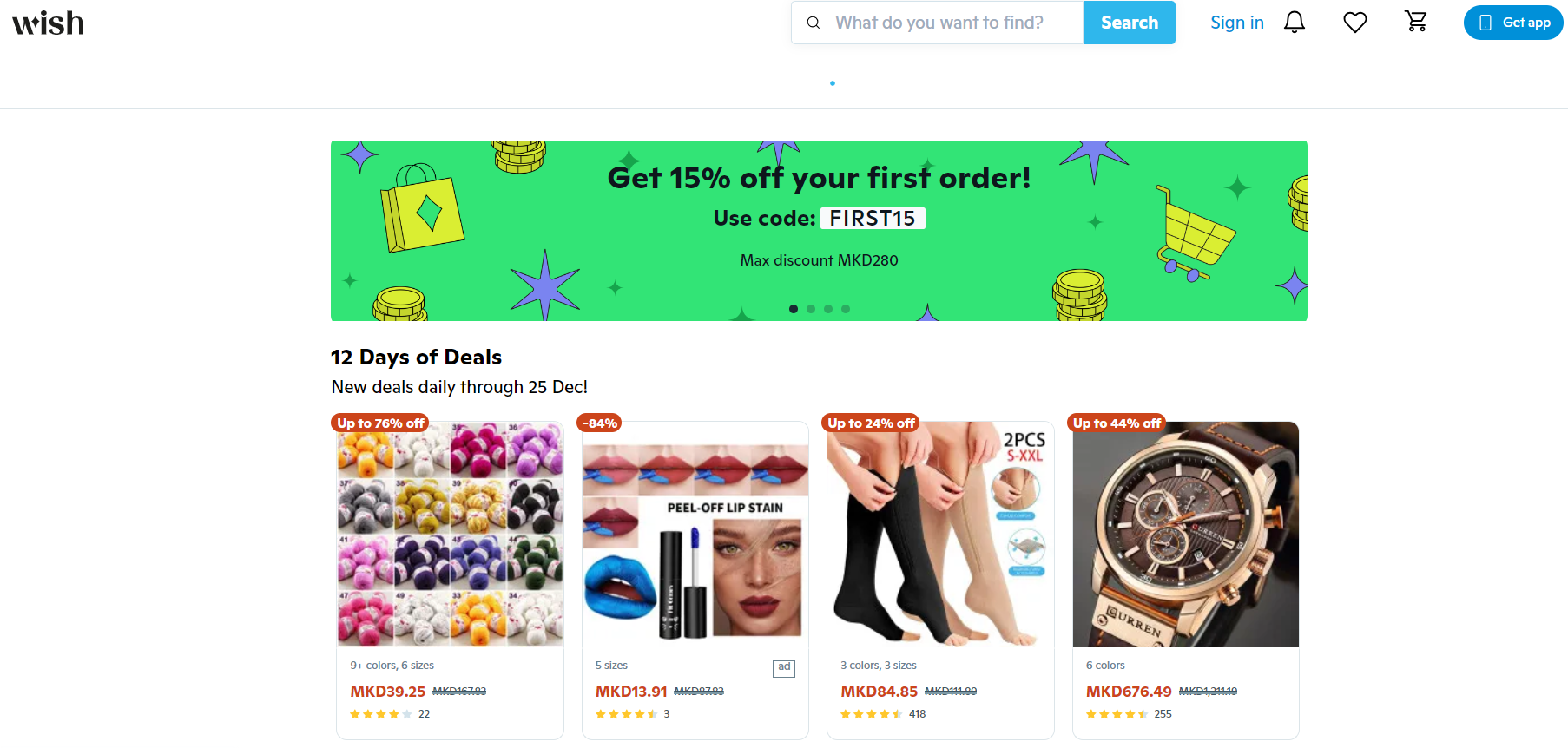The image depicts a webpage from a shopping website identified by the word "wish" in black text at the top left corner. To the right of this, there's a significant blank space until reaching the top center, where a search bar is situated. The search bar contains the prompt "what do you want to find?" and a "search" button in white text on a blue background. Continuing right, there is a "sign in" option in blue, followed by three icons: a bell, a heart, and a shopping cart. At the top right corner, there is a "get app" button in white text within a blue bubble.

Dominating the center of the image, the website displays featured products with a promotional banner on the middle left that reads "12 days of deal" in bold black text. Below this, a lighter text states "new deals daily through 25 December." Four products are showcased in square brackets with their respective prices: the first product priced at MKD39, the second at MKD13.91, the third at MKD94, and the last product at MKD676. The layout accentuates the seasonal deals and facilitates effortless navigation through the site.